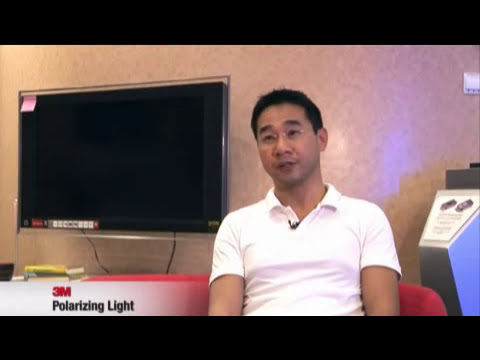The image captures an Asian man with short hair and gold-rimmed glasses seated on a red couch, likely being interviewed. He is shown from the waist up, wearing a white short-sleeved polo shirt with a microphone clipped at the collar. Behind him, a large flat screen monitor is mounted on a light brown patterned wall, showing mostly a black or blank screen with a pink post-it note affixed to it. To the lower left of the image, there is text reading "3M" in red, followed by "polarizing light." The scene suggests the man is discussing a technical topic, possibly related to polarizing light. On the right side of the image, there is an unidentifiable machine, while a podium or informational stand is also visible.